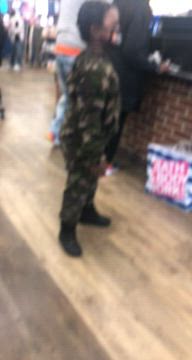In this slightly blurry photograph, a young boy, clad in green fatigue pajamas and short black boots, stands beside an adult woman at a checkout counter inside a retail store. The boy, who has dark skin and short black hair, wears a gold-colored surgical mask. The checkout counter is constructed of red brick with a sleek black countertop. The woman, seen from behind, appears to be opening her wallet. At her feet, a large shopping bag with white and blue stripes and the Bath and Body Works logo in white letters set against a red background lies prominently. She is dressed entirely in black with white shoes. In the background, the store is bustling with other shoppers going about their activities.